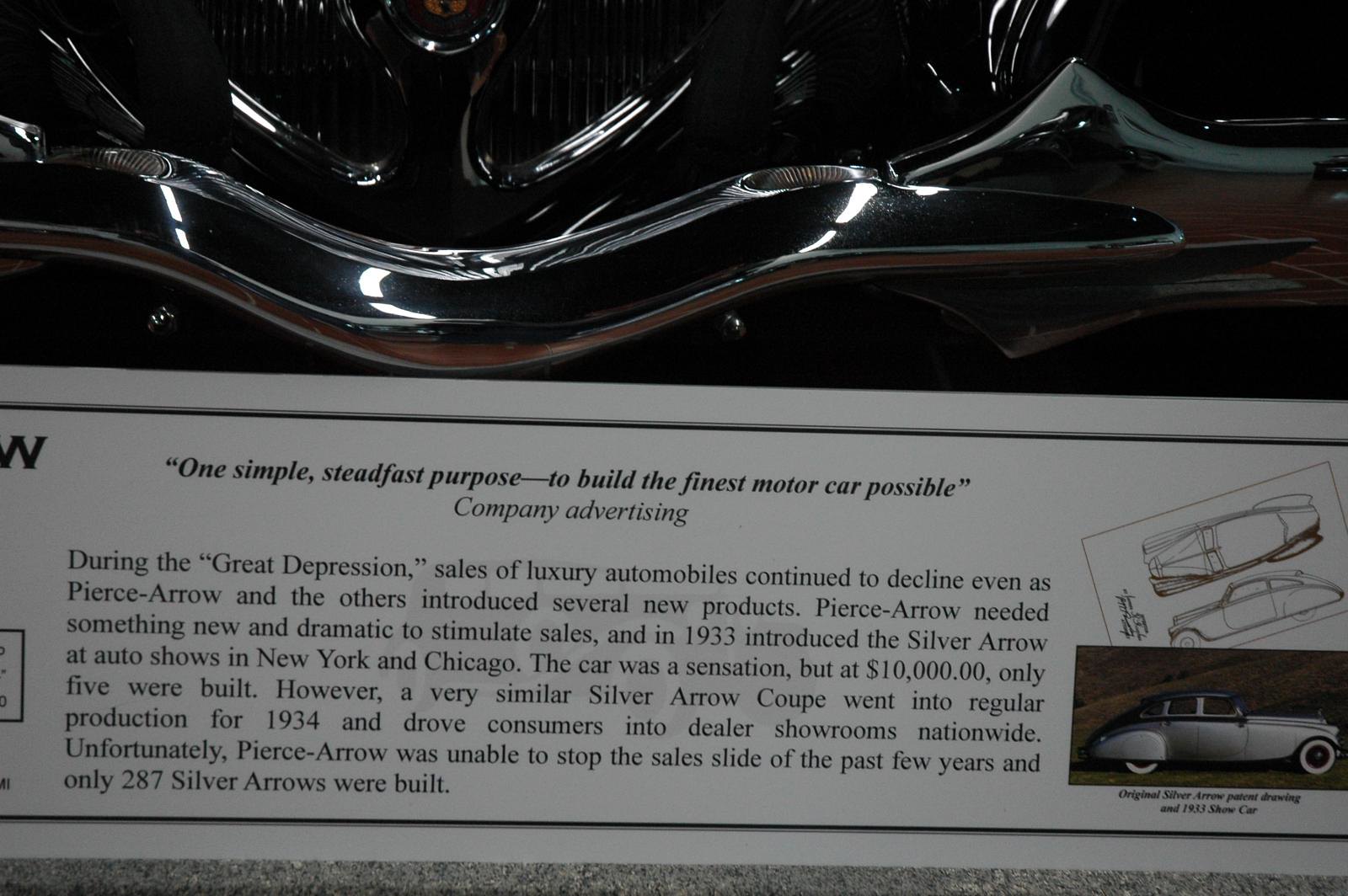The photograph captures a museum display featuring a white rectangular plaque with a thin black border, placed on top of a stone floor. This plaque prominently displays a quotation in black text at the top: "One simple, steadfast purpose, to build the finest motor car possible," attributed to Company Advertising. Below the quote, a detailed paragraph describes the Pierce Arrow company's efforts to innovate during the Great Depression, highlighting how luxury automobile sales declined despite their introduction of new products, including the Silver Arrow. On the right side of the plaque, there is a picture of the "Original Silver Arrow," a patent-pending 1933 show car depicted in a classic 1900s style. In the background of the image, partially in shadow, the chrome bumper and grill of a silver car can be seen, suggesting the presence of the actual vehicle above the plaque, enhancing the museum display's immersive experience.